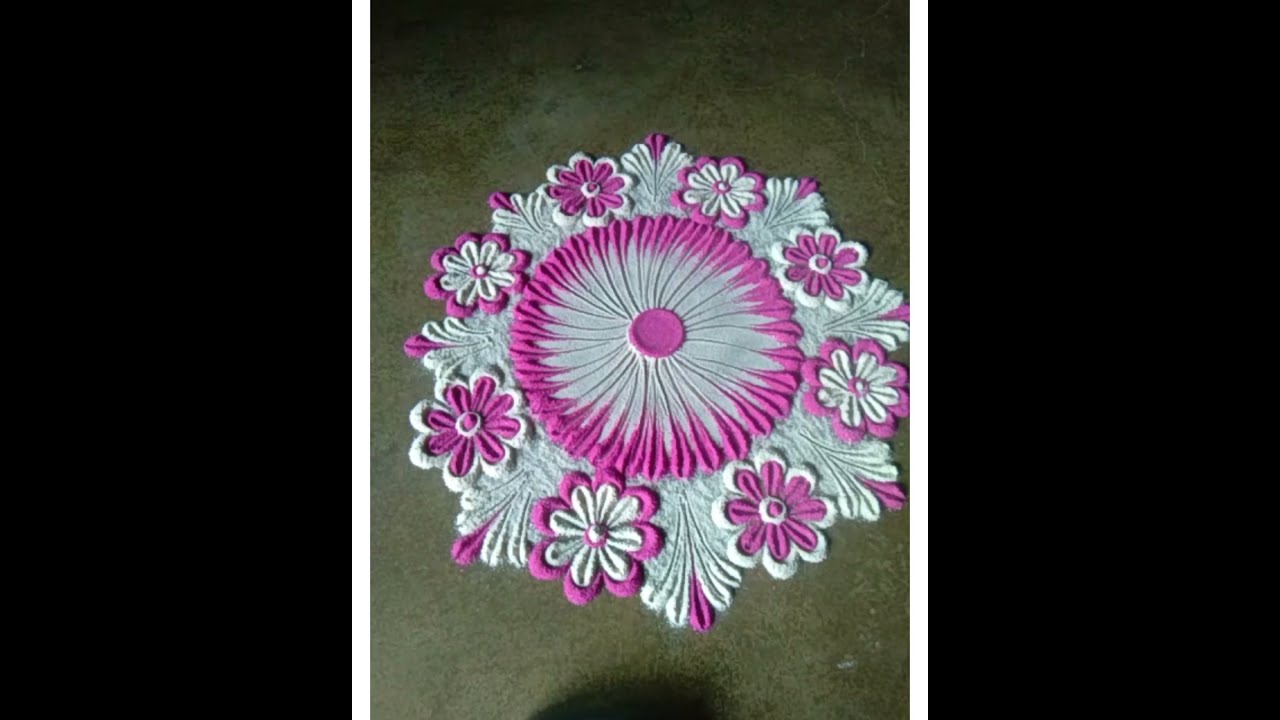This image is a horizontally aligned rectangular photograph featuring a large floral design placed on a green ground, possibly grass. The focal point is a flower-shaped fabric arranged in a detailed, symmetrical pattern. The fabric is predominantly white, adorned with alternating floral patterns: one being white with pink edges and the other pink with white edges. These flowers are arranged in a circular formation around a central pink circular spot. This central spot is surrounded by a white area, which is further encircled by pink details, creating a layered effect. The design resembles a doily, with flowers separated by curved lines between them. Additionally, the photograph includes thin vertical white borders on the left and right sides, enclosed by solid black vertical strips. The intricate floral design stands out prominently against the green backdrop, emphasizing the delicate interplay of white and pink colors.